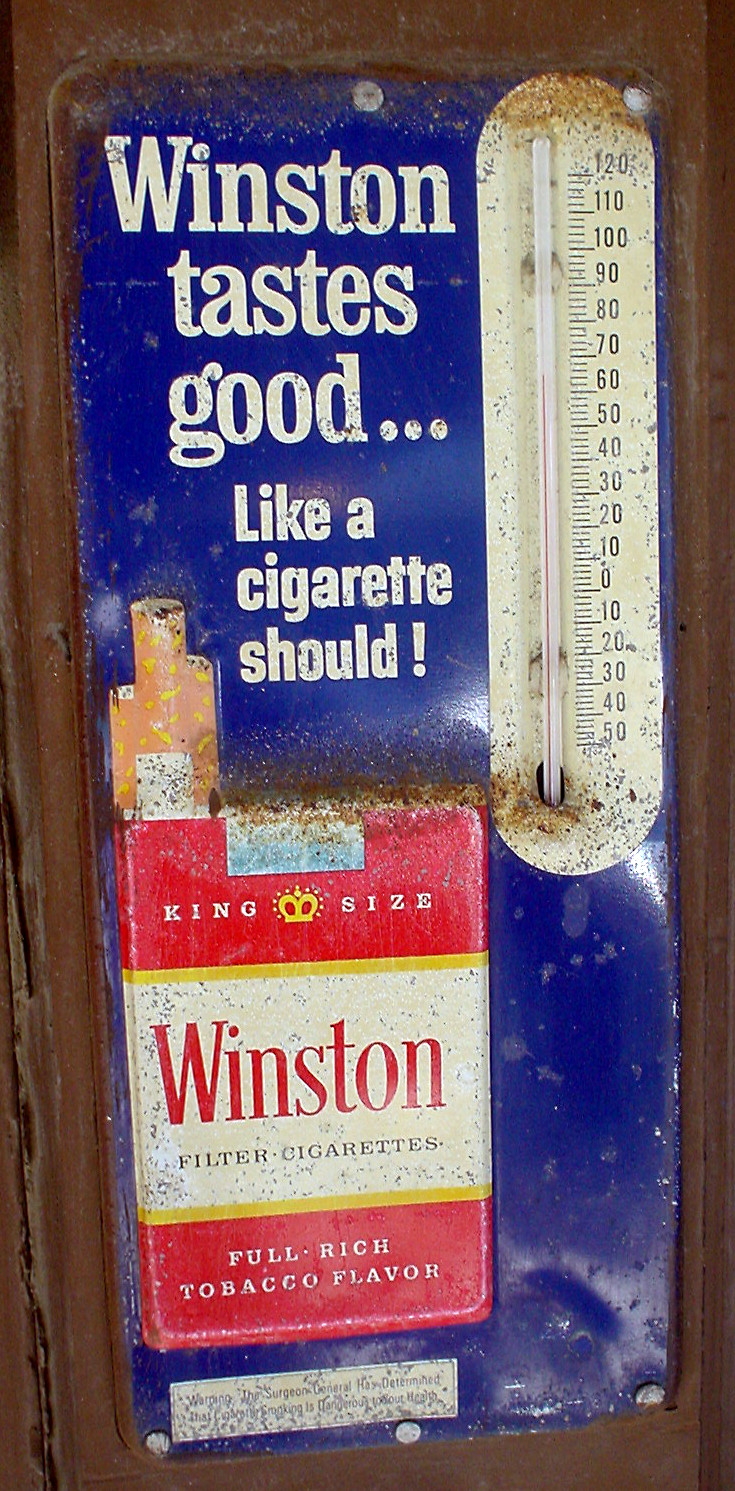A vintage tin sign advertising Winston cigarettes is prominently displayed, featuring both an integrated thermometer and considerable signs of aging. The sign's primary background is a timeworn blue, contrasted by bold white text proclaiming "Winston Tastes Good Like a Cigarette Should." Below this tagline, there is a detailed depiction of a red, white, and yellow Winston cigarette pack, indicative of a soft pack with three cigarettes partially emerging from the top. The cigarettes are illustrated with distinctive brown filters and white paper. This pack prominently displays the words "Winston Filter Cigarettes, Full Rich Tobacco Flavor," with "King Size" written above in red letters accompanied by a yellow crown symbol.

The entire sign shows significant wear: the edges are dented, the colors are fading, and patches of rust are spread across the surface, emphasizing its age and exposure to the elements. The thermometer, calibrated in Fahrenheit, ranges from -50 to 120 degrees. The sign appears to be affixed to a dilapidated metal shed, itself rust-colored and evocative of a bygone era.